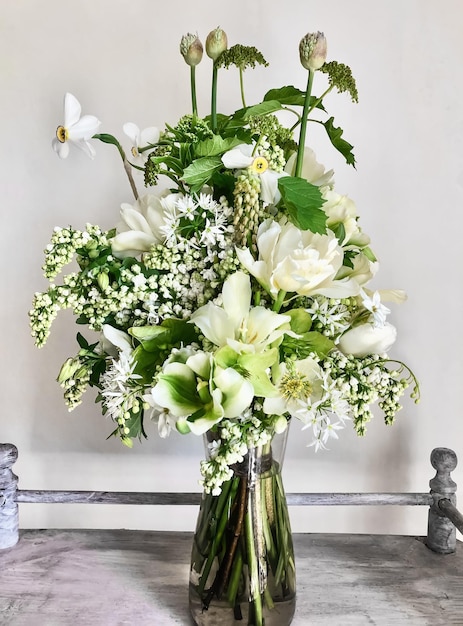In the foreground of the image, there's a transparent glass vase filled with water and a vibrant bouquet of white and light green flowers, reminiscent of a wedding arrangement. The vase reveals the stems and water level inside, while the bouquet itself consists of a variety of small and large blooms, along with sprigs of tiny flowers and green leaves. Tall white flowers extend upward and slightly to the side, creating an elegant, multi-dimensional display. This vase sits on a grey table or trolley, which features a border resembling a little fence made of interconnected vertical and horizontal steel rods. The setting is simple, with an off-white wall in the background, casting a faint shadow of the table and vase.